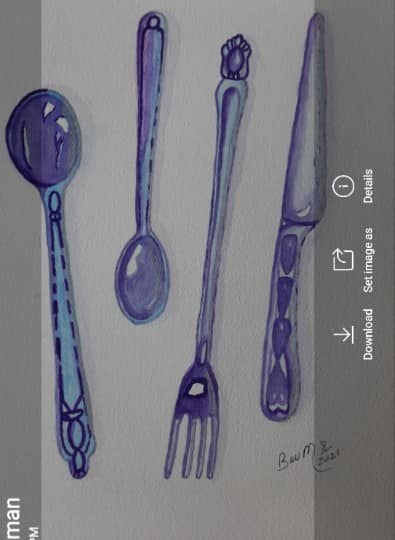This detailed image is a screenshot capturing a highly realistic and meticulously drawn depiction of blue cutlery. The drawing is presented on a white rectangular background with gray borders. The cutlery includes two spoons facing different directions, a fork pointing downward, and a butter knife pointing upward. The utensils feature a strikingly clear blue color with intricate shading and reflections that give them a three-dimensional appearance. Their handles are adorned with elaborate stencils and elegant designs, enhancing their visual appeal. On the right side of the image, mobile phone icons for "download," "set image as," and "details" indicate it is indeed a screenshot. At the bottom right, a partially legible signature reads "BAUM" and possibly "2021," hinting at the artist's name and the year of creation.